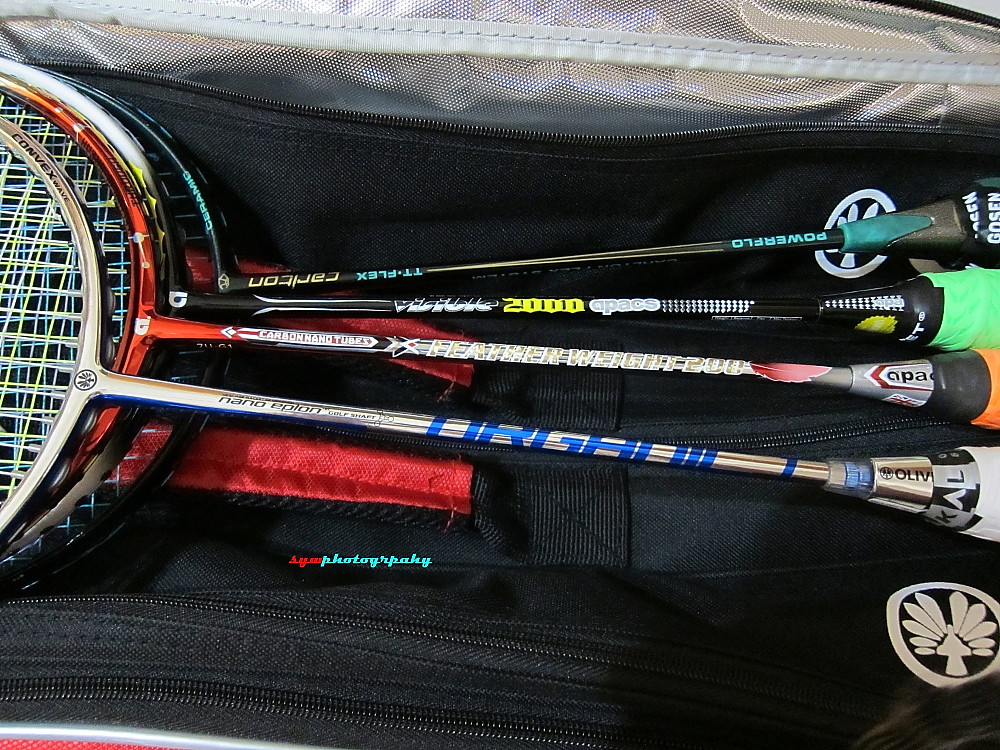The image features a collection of four badminton rackets neatly organized within a black carrying case, which is adorned with a logo of a white turkey in the bottom right corner and a watermark that seems to read "SYW Photography," though there's a typo with the letters 'P' and 'A' swapped. The case has a silver-lined interior at the top and black zippers. Each racket is identifiable by its distinct branding and color scheme. From top to bottom, the rackets exhibit a variety of labels such as "Nano" in blue lettering on a silver pole, "Featherweight 200 Carbon Hand Tubes" in gray and red, an unreadable brand with "2000 Apex" on a black pole, and "Powerflow TT Flex Caricon" on another black pole with a neon green handle. The netting of the rackets is consistently yellow and blue, and they are stacked so the netted parts are aligned to the left side of the image, while the handles, in neon green, orange, white, and black, are displayed to the right, giving a clear view of their lengths and colors. The detailed alignment and distinct coloration of each element contribute to the orderly yet vivid depiction of the badminton equipment.